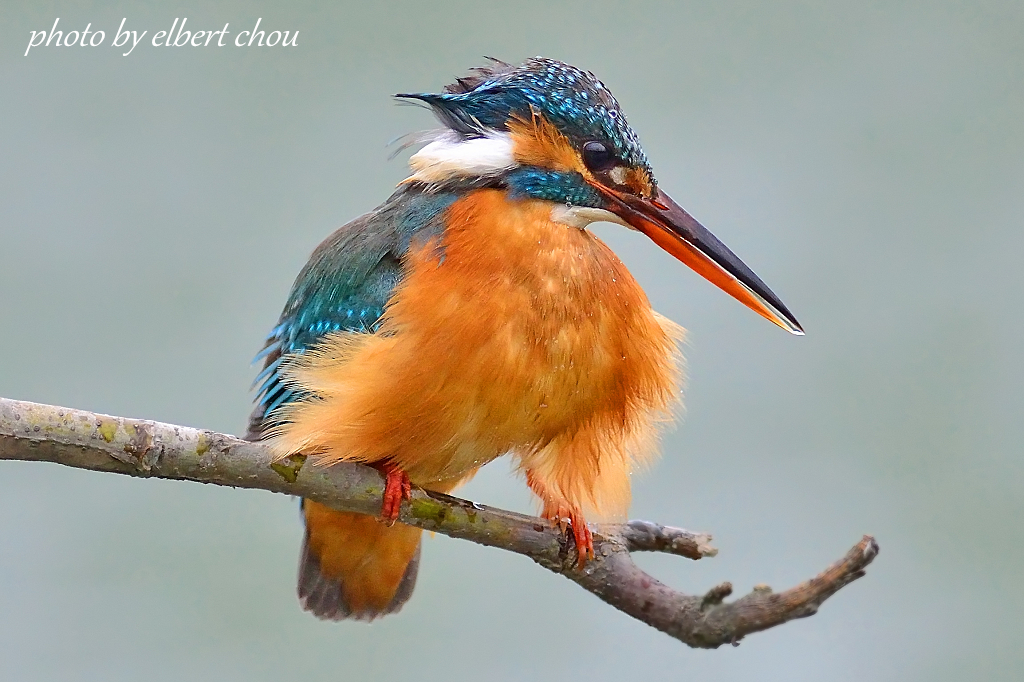In this detailed photograph taken by Albert Chow, prominently credited in white italic font in the upper left corner, a small but striking bird is captured sitting on a slender branch. The background is a blurry gray, making the bird the focal point of the image. The bird is turned to the side, showcasing its visually captivating plumage. Its head is adorned with blue, speckled feathers, complemented by dark eyes. The bird's beak is notably long, resembling that of a pelican, with the upper part being dark and the lower part a bright orange. The neck area is encircled by white feathers, which continue to the back of the head. The upper part of the bird's back showcases more blue feathers, some with intricate dots, while the rest of the body transitions into a vibrant orange hue. The bird's feet are a striking, vibrant orange, adding an additional splash of color to its elegant appearance. The fine details and vivid colors of the bird contrast beautifully with the subtle background, making this photograph a stunning portrayal of nature.